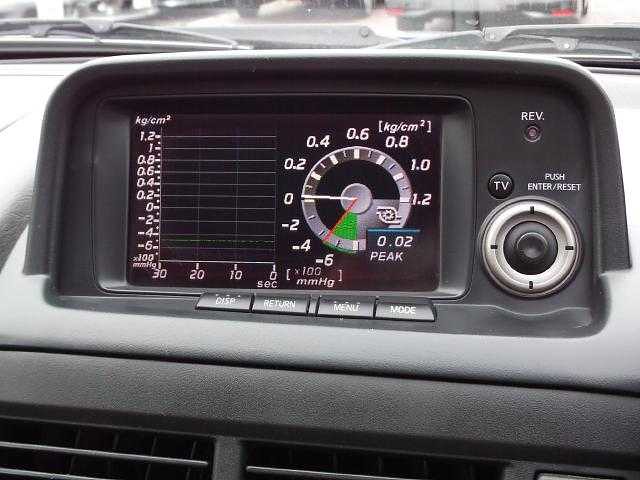This image captures the detailed view of the central console area of a car, showcasing various controls and displays. Dominating the center is a black screen featuring a detailed gauge marked "KG/CM2." The circular gauge has increments of 0.2, ranging from 0 to 1.2 on the top half, and descending to -6 on the bottom half. Notably, a white line points towards zero and a red line appears past -4, accompanying a green section. Additionally, there’s a small box displaying "0.02 peak."

Adjacent to the screen are several tactile controls. To its side, there are buttons labeled "Rev," in red, a black button marked "TV," and another button inscribed with "Push, Enter/Reset." Below these controls is a textured silver wheel with a black button at its center. Further down, another array of buttons is visible, marked respectively as "DISP," "Return," "Menu," and "Mode."

The console also exposes a portion of the car's air conditioning vents, and a glimpse beyond the confined interior reveals the windshield wipers, dashboard, and part of the exterior with other parked cars visible through the windshield. This comprehensive view highlights the intricate instrumentation and user interface designed for modern vehicle operation and information display.